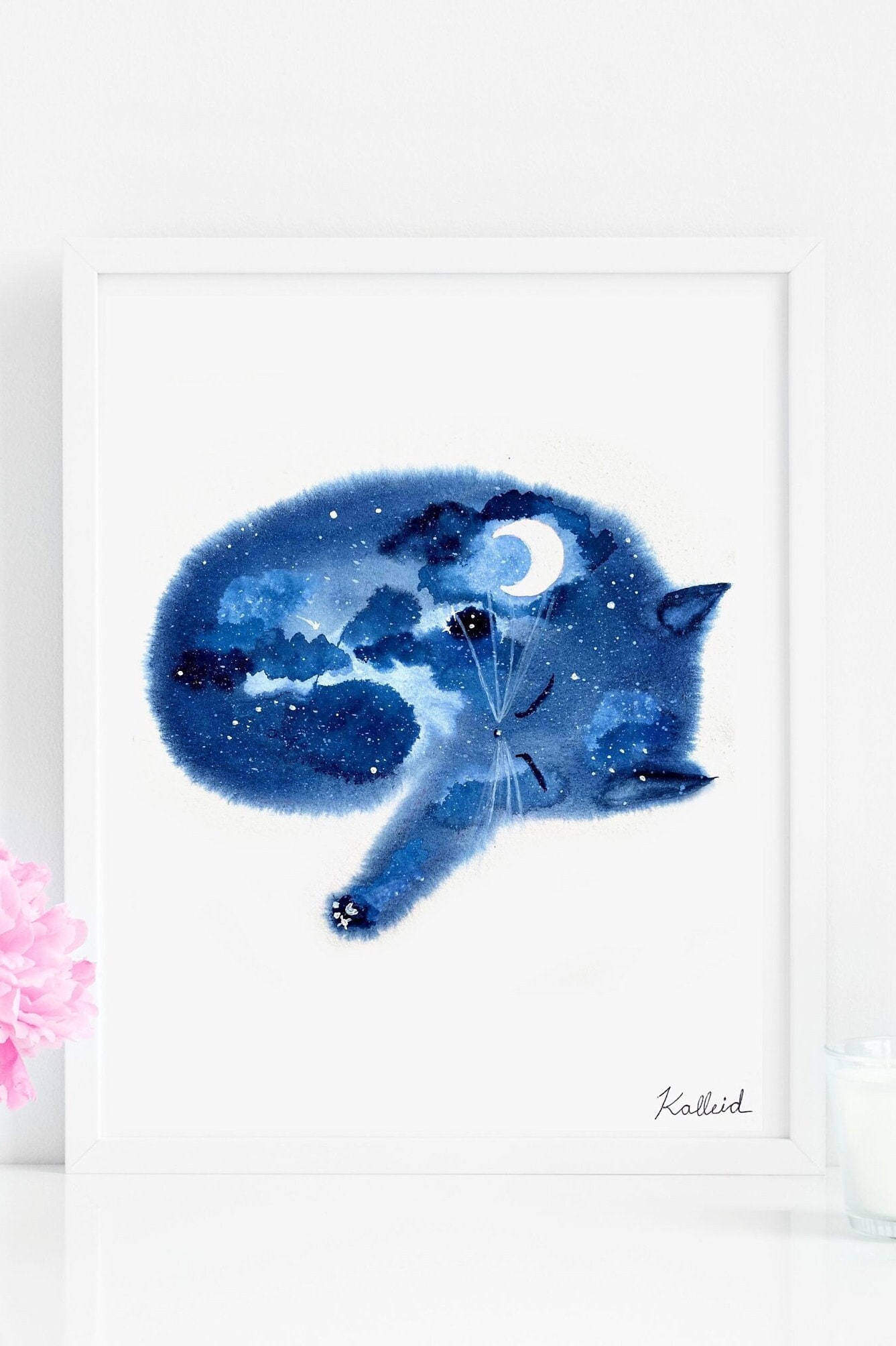This captivating artwork features an abstract, watercolor painting of a blueish cat that appears semi-transparent, curled into a ball with its left paw extended towards the viewer. The painting, which resides on a white canvas and is framed within a gray border, is set against a white background. A partial pink flower peeks in from the left side of the frame, adding a touch of color contrast. Artist Khalid, or possibly "Kallied," has signed the piece in the bottom right corner. The cat embodies the night sky, with elements like fluffy clouds, dark trees, and a prominent crescent moon intricately integrated into its fur. The moon’s shadow can even be perceived in the cat’s ears, making this artwork a stunning blend of feline and celestial elements.